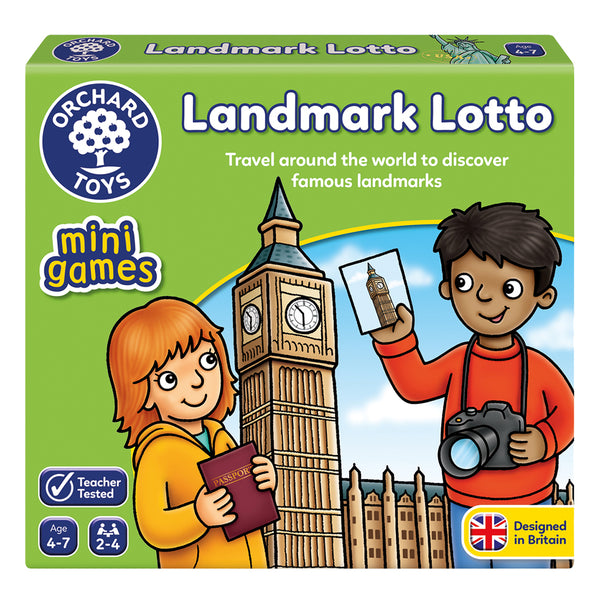The image features a brightly colored box of a children's toy game called "Landmark Lotto." The top of the box displays the game’s title in white text with blue outlines, and the overall box color is green. The game is produced by Orchard Toys, whose logo—a white-colored text with a tree illustration—appears in the upper left corner. The word "minigames" is written in yellow on the left side.

The bottom of the box includes several labels: one stating "teacher tested" with a checkmark, another indicating the appropriate age range "4-7," and a note that the game is designed for "2-4 players." On the right side, a label in blue text under a yellow banner declares that the game was "designed in Britain," accompanied by a partial image of the British flag.

The front design showcases a cartoon scene where a boy with dark brown skin and fluffy black hair, wearing a red sweater and blue jeans, holds up a card depicting Big Ben. He has a smiling expression, bright eyes, and a black camera hanging around his neck. Beside him is a shorter girl with reddish-orange hair, a yellow jacket over a blue undershirt, and a bright, cheerful face. She holds a passport-style book and looks at the card the boy is displaying. The scene emphasizes travel and discovery, fitting the game’s educational theme of exploring famous landmarks around the world.